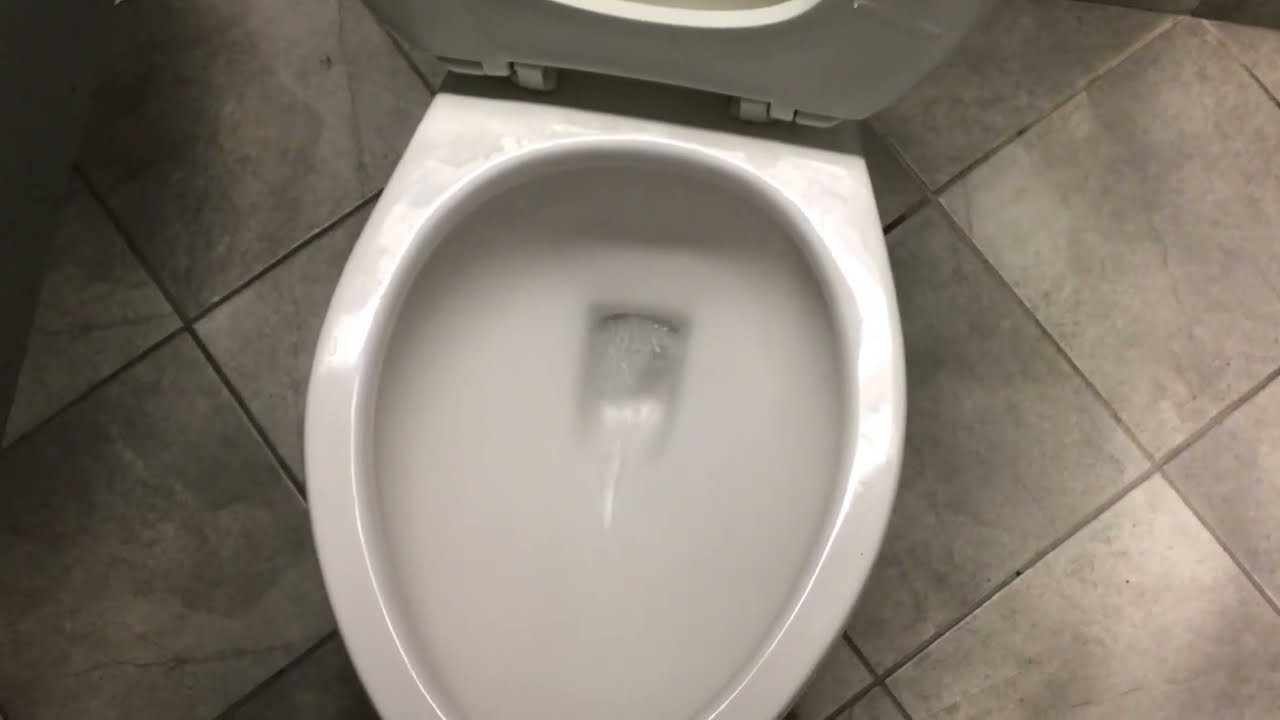The image depicts a clean, spacious bathroom with a grayish marble tile floor. Dominating the scene is a white porcelain toilet with the lid up, slightly angled in the center of the photograph. The light, coming from the right, casts a glow on the toilet while leaving the left side of the image darker in comparison. The toilet appears to have just been flushed, as there are bubbles and water movement visible within the bowl. The overall color palette of the bathroom includes shades of gray, white, and hints of brown and black, contributing to a modern, pristine look that suggests this might be a public restroom. The floor appears immaculate, further enhancing the clean and orderly atmosphere of the space.